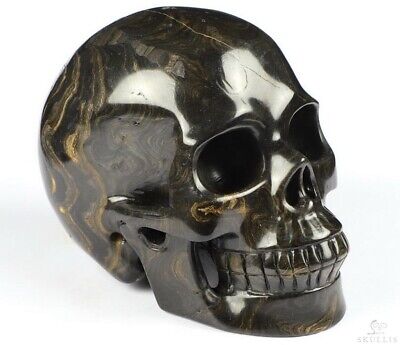This image features a professionally photographed, highly detailed decorative skull, likely made of a shiny black stone or ceramic material, possibly resembling black quartz or marble. The skull is intricately carved to emulate a human skull, complete with eye sockets, nasal cavity, and a full set of teeth, which creates a semblance of a smile. Subtle golden or yellowish swirls and veins are dispersed throughout the surface, more prominently at the back, enhancing its luxurious appearance. The skull is viewed in a three-quarter angle, allowing a clear view of its profile as well as the front. A subtle reflective shine suggests a smooth, polished finish, and a signature, albeit partially unreadable, can be seen to the right of the image.